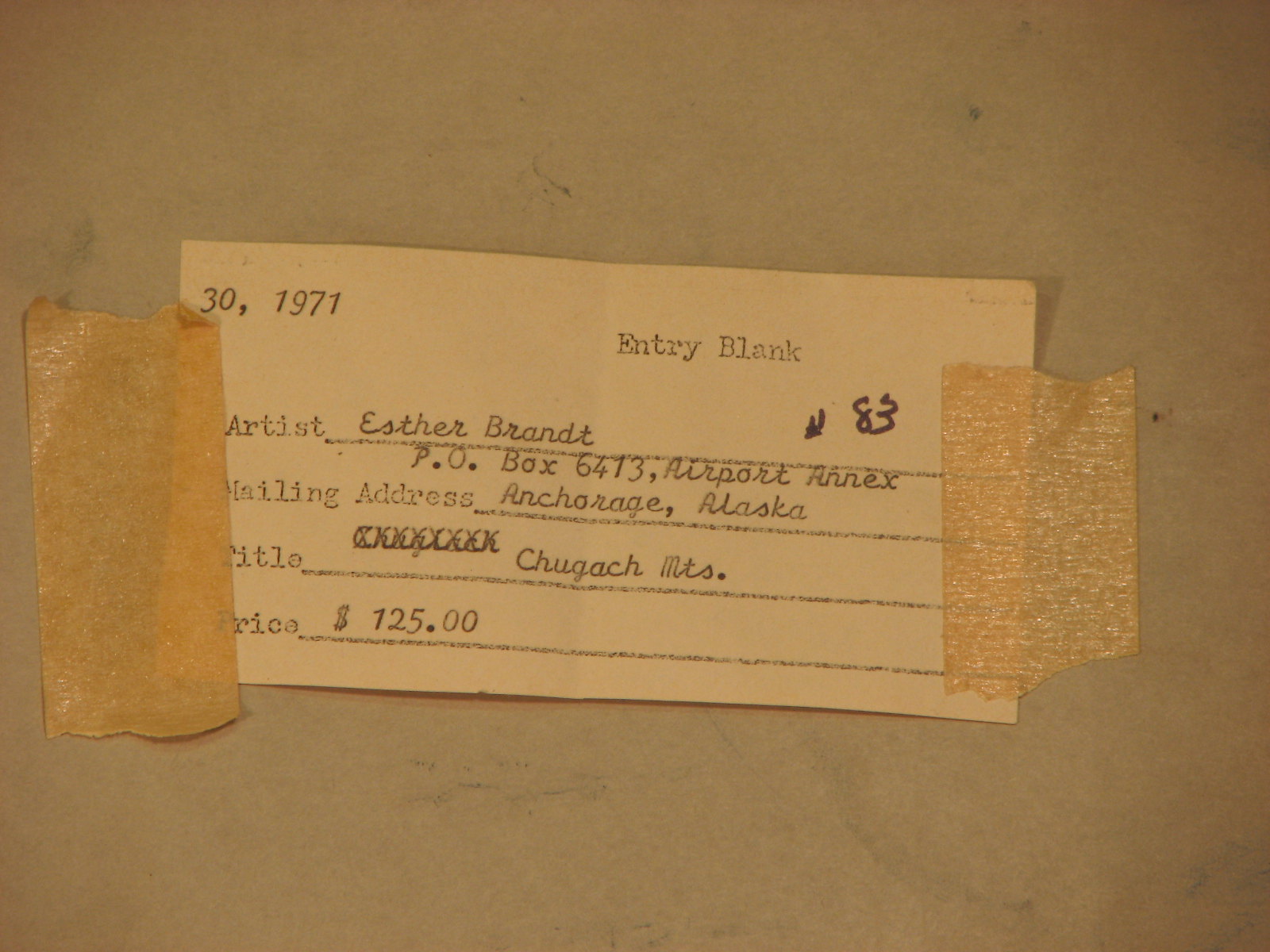This image is a photograph of a yellowed and creased index card, likely from 1971, used to label an artwork for sale. The card has been taped to a brown, cardboard-like surface using two pieces of masking tape. At the top, it is labeled "entry blank" and includes various fields filled in with typed and handwritten details. The artist is Esther Brandt, her mailing address is P.O. Box 6473, Airport Annex, Anchorage, Alaska, and the title of the artwork is "Some Mountains." The price of the artwork is listed as $125. The number 83 is also handwritten on the card.